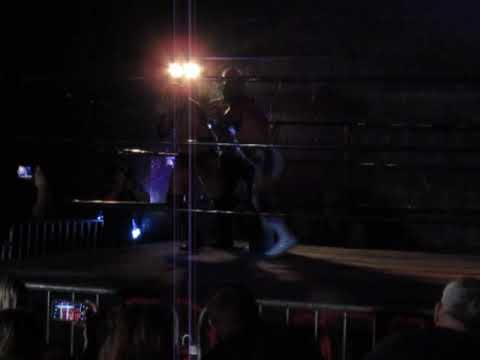This photograph captures a dimly lit indoor scene, possibly from a nighttime event or concert. The central focus lies on a stage or platform made of wooden planks, set against a backdrop of a brick wall. On this stage, there are two figures who appear to be engaged in a fight, reminiscent of a wrestling match, though their actions are somewhat blurred due to the darkness. The stage is dimly illuminated by two bright lights and accented by subtle purple lighting, while the ropes surrounding the stage are black, indicating a wrestling ring-like setting.

Surrounding the stage, there's a crowd of spectators positioned behind metal barricades. Some members of the audience are visible, with notable details like a person with gray hair or wearing a hat in the bottom right corner. Adding to the scene's dynamic nature, a few spectators can be seen recording the event with their mobile phones, capturing the intense engagement on stage. The overall ambiance suggests a lively gathering where the audience is actively involved in the spectacle unfolding before them. The photograph's color palette includes shades of black, light blue, light purple, yellow, gray, red, and blue, contributing to the event's vivid yet dark atmosphere.